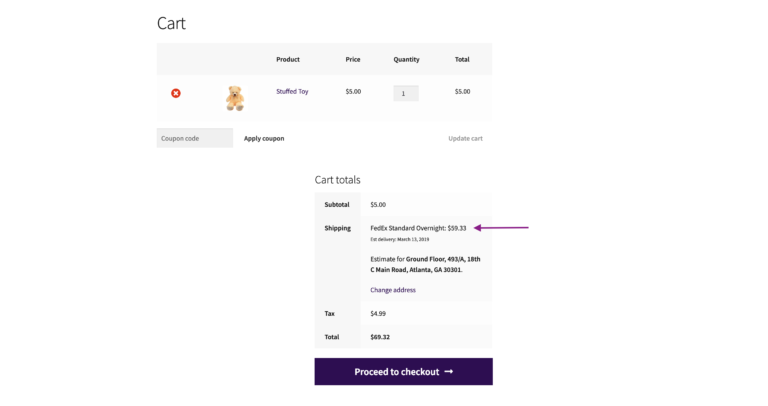This image is a screenshot of a shopping cart interface, predominantly featuring a white background. The cart includes a single item: a light tan-colored stuffed bear toy. At the top, the word "Cart" is displayed. Below it, there are grayed-out sections designated for product price, quantity, and total.

The interface has a small "X" icon allowing users to remove the item from the cart. The stuffed toy is named "Stuffed Toy," and it's hyperlinked for more details. The price of the toy is $5.00. The entered quantity is 1, bringing the total to $5.00.

Beneath the item details, there is a field to enter a coupon code, accompanied by an "Apply Coupon" button. To the right, there's an option to "Update Cart."

At the bottom right of the interface, the "Cart Totals" section displays the subtotal of $5.00. Below it, there's information about shipping options with FedEx Standard Overnight costing $39.33 and an estimated delivery date of March 13, 2019. The shipping address is listed as 439-A, 18th C Main Road, Atlanta, GA 30301, with an option to change the address via a purple link. 

The tax is calculated at $4.99, resulting in a grand total of $49.32. At the bottom, there's a prominent purple button labeled "Proceed to Checkout."